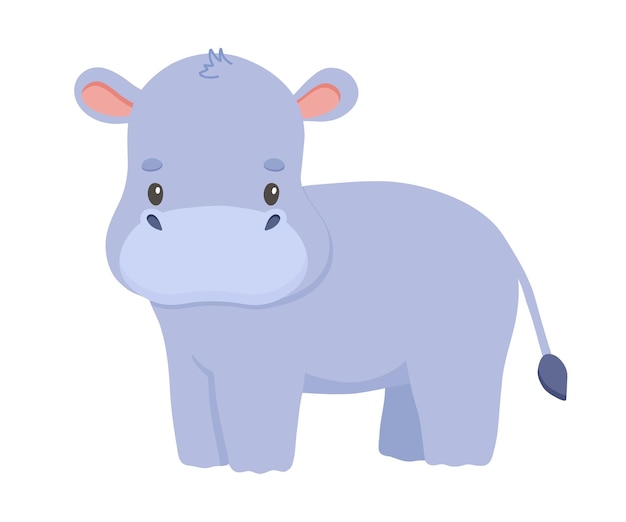This image depicts a whimsical cartoon version of a hippo, primarily light blue with shades of deeper blue and hints of black shading. The hippo has a distinctive dark blue tail with a small cotton-ball tip, adding to its playful appearance. Large floppy ears, blue with pink interiors, frame its small, black-dotted eyes, which contribute to the hippo's minimalist, slightly expressionless face. It has no visible mouth, small nostrils, and tiny eyebrows, embodying a simple yet endearing design reminiscent of a children's book illustration. The hippo's feet are rendered as blue stumps, with subtle indents suggesting toes. A tuft of hair sits atop its head, adding to its charm. The entire scene focuses solely on the hippo, emphasizing its cartoonish, almost cow-like form with its head turned forward to face the viewer while its body is shown in profile.